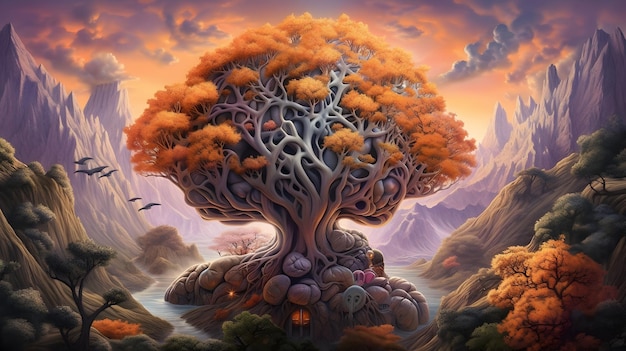This digital artwork features a majestic, large tree prominently centered in a fantastical landscape. The tree, with its intricate structure of intertwining branches, culminates in a dense tuft of orange and auburn leaves, forming a circular canopy. Below the tree, which stands majestically as if rooted in a rocky terrain, there's a door-like structure nestled under its sprawling roots, and rocks surround this base. Flowing gently around these roots is a stream that splits and meanders to either side of the tree, eventually fading into the land.

This scene is set against a dramatic background of towering, grey rock mountains flanking both sides, with golden hues peeking through. The mountains add a sense of grandeur and mystique to this surreal setting. The sky above is awash with rich, orange and purple hues, suggesting either a sunrise or sunset. Wisps of clouds stretch across this vivid sky, adding to the atmospheric depth. Large, prehistoric-looking birds soar through the air on the left side, heading towards the viewer.

In the bottom right, a smaller, singly colored tree contrasts with the dominant central tree, while to the bottom left, there are green and auburn shrubs, providing a lush undergrowth. Scattered throughout the scene on both sides of the river are various green and orange trees, enhancing the vibrant, yet harmonious color palette of the artwork. The detailed, almost futuristic aesthetic of the image evokes a sense of otherworldly wonder.